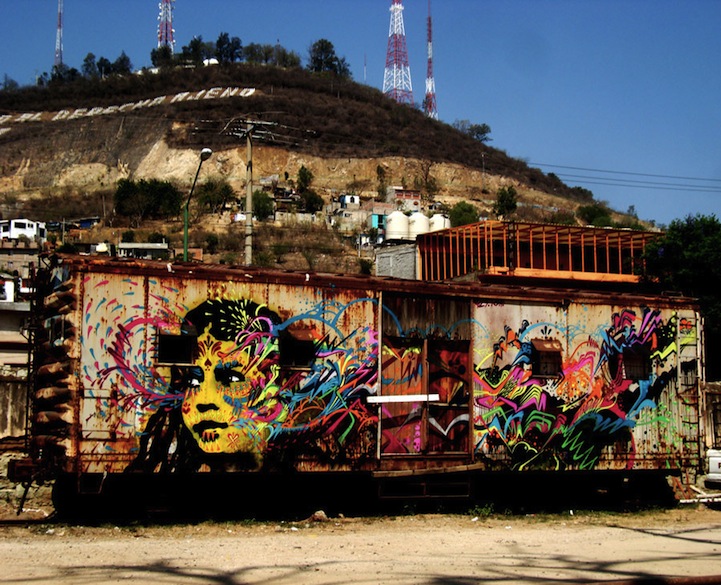The image depicts a daytime outdoor scene characterized by a large hillside or mountain that extends from the left-hand side toward the right. The hillside, which features a mix of bare dirt and dried grass, is topped with several prominent structures, including red and white radio towers and antennas. Scattered among the hillside are some houses and a few trees with green leaves. Written words, seemingly in Spanish, are visible on the hillside, though they are difficult to discern.

At the base of the hill, running parallel to a dirt road and parking lot, are train tracks situated in an industrial area. Alongside the tracks lies an old, rusted rail car that appears abandoned. This rail car is adorned with vibrant and intricate graffiti, showcasing a mural of a girl's face in shades of blue, pink, yellow, and green, with additional scribbles and lettering. The scene also includes various utility elements, such as power lines and industrial tanks. Cars are visible traveling on the road near the rail car, further highlighting the urban-industrial setting.